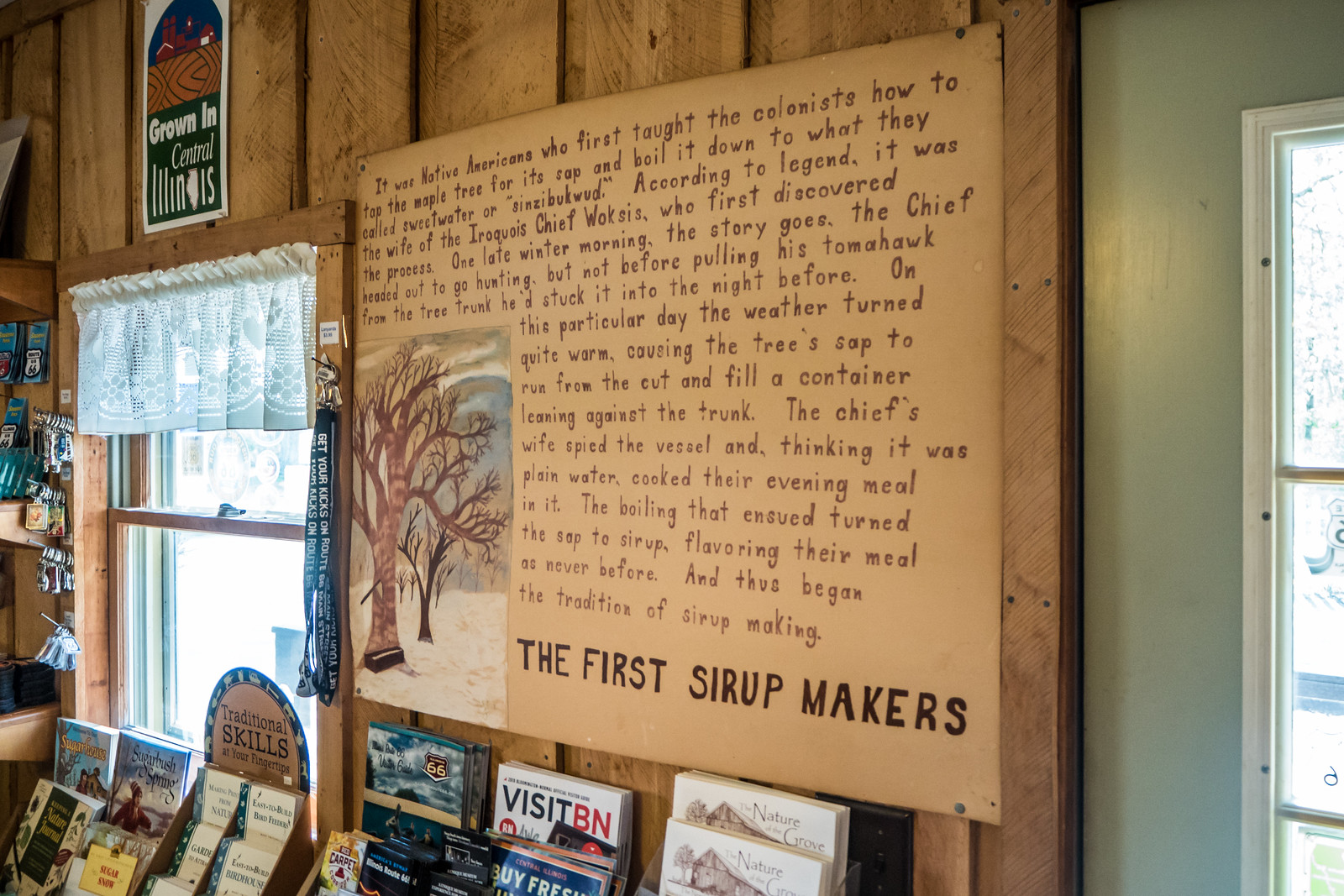The image depicts an indoor scene, likely within a library or a bookstore. The main wall is constructed of light-colored wooden planks, adding a rustic charm to the interior. Prominently displayed on the wooden wall is a large, old-school poster with a depiction of trees in a snow-covered landscape. The poster narrates the legendary origins of syrup making, detailing how Native Americans taught colonists to tap maple trees and boil the sap into syrup, with an illustrative tale involving the Iroquois chief Woxus and his wife. This legend is detailed in a textual paragraph on the poster, which concludes with the phrase, "The first syrup makers" in bold black letters.

Beneath the informative poster, there is a wooden shelf lined with various magazines. Adjacent to this is a window with a wooden border featuring small clear curtains, letting in daylight. Hanging from nails on the window sill are lanyards and keychains. The left side of the room showcases several bookshelves filled with diverse reading materials, including children’s books on traditional skills such as building bird feeders and houses, and nature-themed titles like "Sugar Bush Spring," "Sugar House," and "Sugar Snow." Another section of the bookshelf displays books on local topics, such as "Visit BN," "Buy Fresh," and "Illinois Route 66."

Overall, the ambiance is cozy and inviting, emphasizing educational and historical themes enriched by detailed narratives and naturalistic visuals.